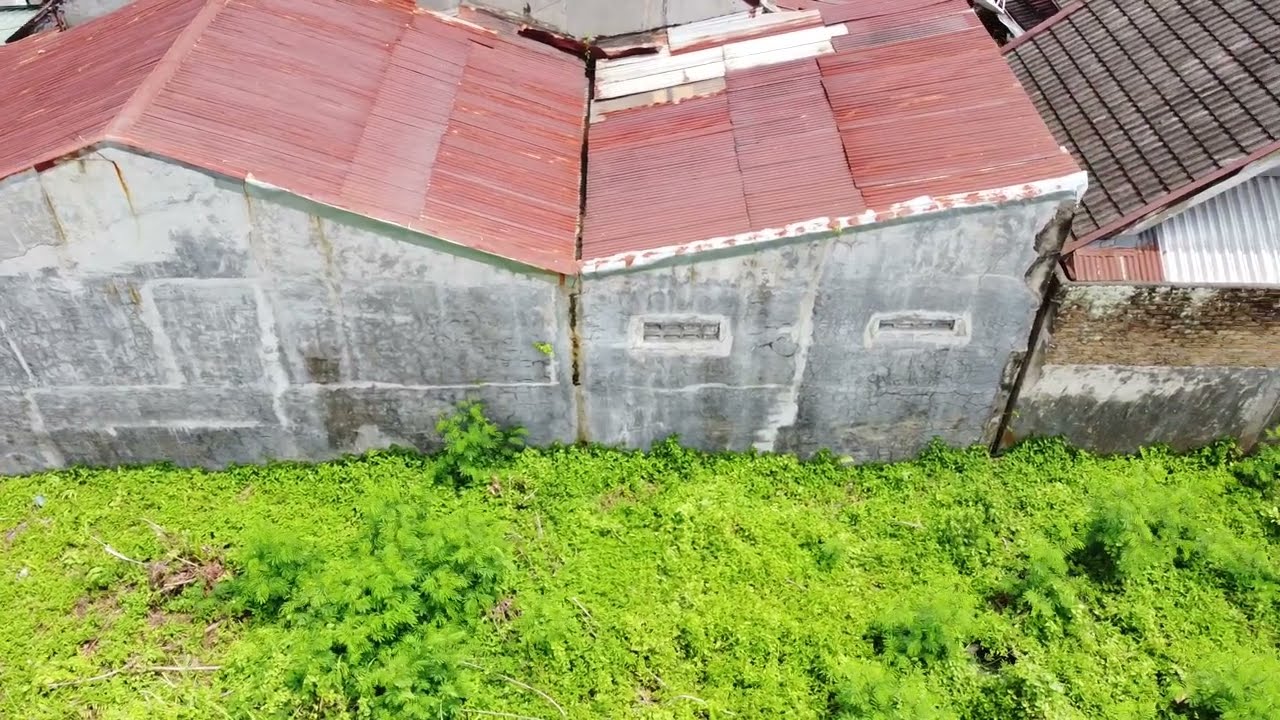This aerial photograph, taken from a drone about 20 to 30 feet above the roofline, depicts an old, dilapidated farm setting on a bright, sunny day. The image captures a large, overgrown field filled with weeds and bright green shrubbery, dotted with small evergreen saplings. Dominating the scene are three large, worn-down buildings nestled closely together. The foremost structure, characterized by its concrete sides and a rusted, red metal corrugated roof, shows signs of aging and repair with patched white plastic panels. Adjacent to it, there is another old building, possibly a farmhouse, featuring a brown tiled slanted roof and a mix of brick and concrete walls. Both structures, situated on what appears to be a farm extension for housing livestock, evoke a sense of antiquity and neglect. The overall atmosphere is accentuated by the vivid contrast of natural greens against the muted tones of the weathered buildings.